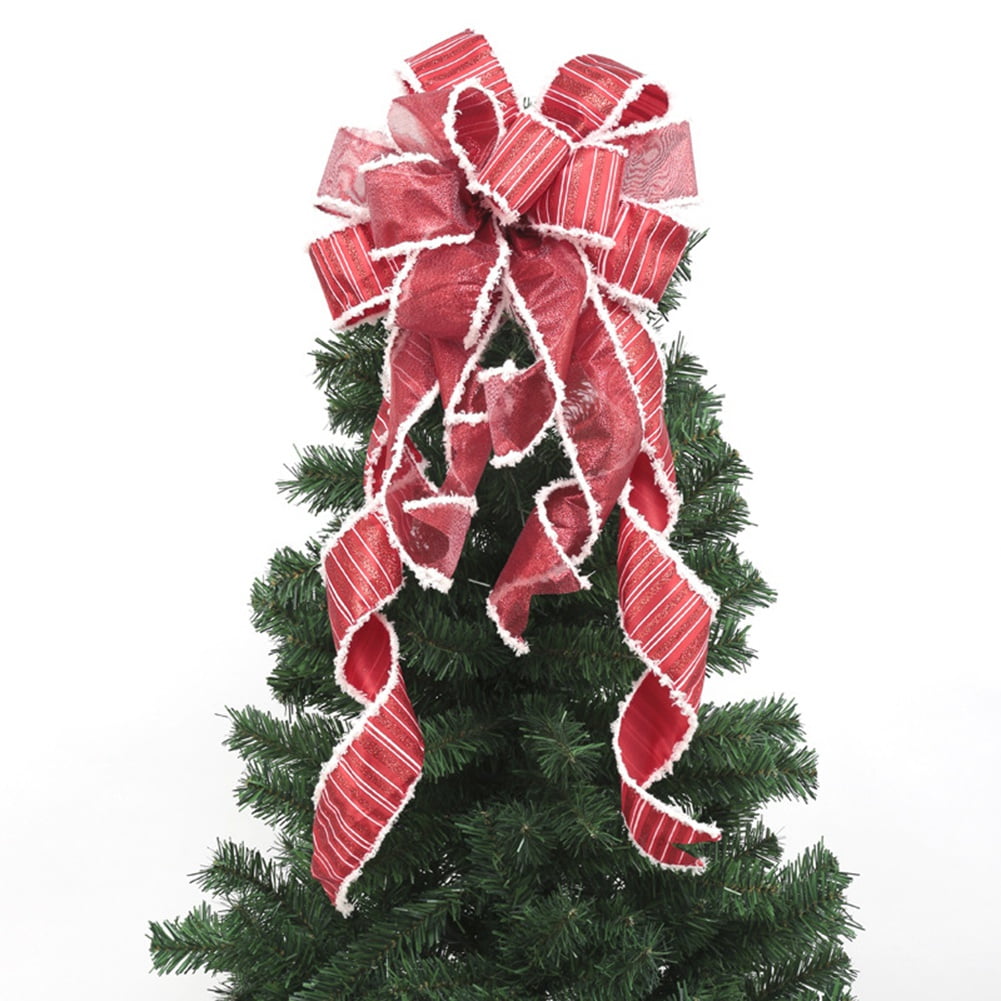This color photograph captures the upper section of a green, artificial Christmas tree adorned with a striking red ribbon. The ribbon, tied into a flower-like decorative bow, features white stripes and white frilly edges, with parts of it gracefully hanging below. The detailed and distinctive ribbon stands out prominently against the otherwise plain white background. The tree, reminiscent of a blue spruce with its medium-sized needles, is captured against an entirely white backdrop, emphasizing the festive decoration.